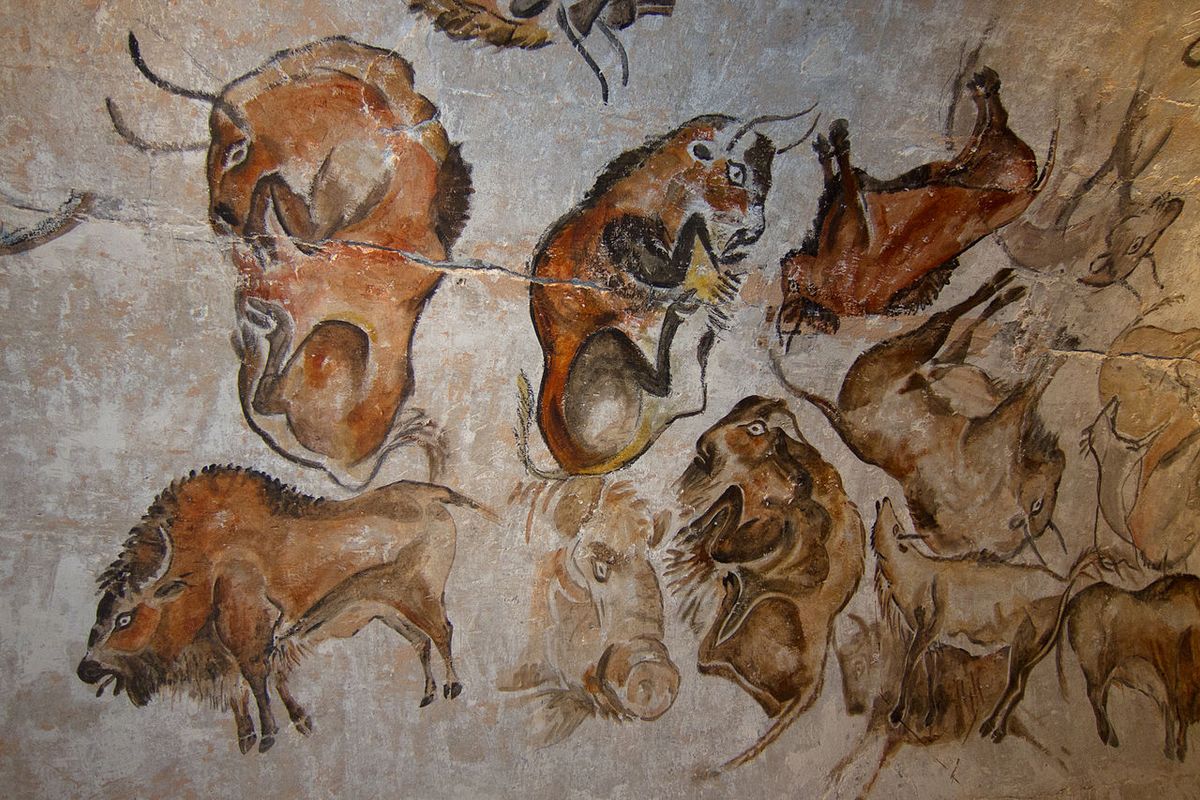The image depicts a weathered, faded drawing on a light grayish, or whitish, stone background, resembling ancient cave art. A prominent crack runs horizontally from the upper left to the lower right of the artwork. The drawing illustrates a variety of large brown mammals, mainly resembling buffalo or bison, characterized by their black faces, black or white horns, four legs, short tails, and bristly backs. The animals are depicted in several positions: standing on all four legs, lying on their sides, curled into fetal positions, or showing close-ups of their heads. They appear in different shades of brown, from dark vivid hues to lighter, faded tones, forming an overlapping collage. Some animals are upside down, adding to the complex and detailed arrangement. The illustration captures the textured detail and intricacy of the ancient art style, with at least 11 or 12 creatures filling the space around the central crack in the stone.